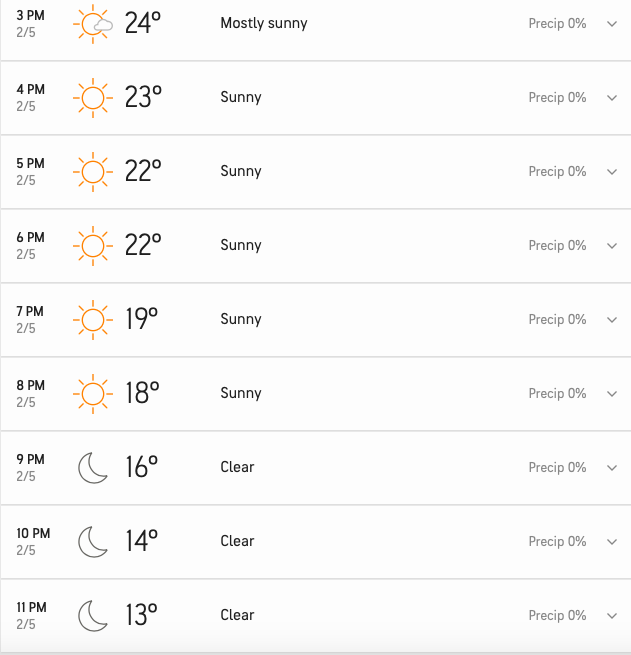This screenshot captures a detailed weather forecast page, providing an hour-by-hour breakdown of the weather conditions from 3 PM to 11 PM. The layout is structured into nine rows, each representing a specific hour within the time range. Each row includes the following elements, from left to right: the time of day at the top, the date beneath the time, an icon depicting the weather condition (such as sunny or cloudy), the temperature in degrees Celsius, a textual description of the weather (whether it's mostly sunny or clear), the chance of precipitation presented as a percentage, and a drop-down arrow which likely reveals additional details.

At the very top of the screenshot, the weather forecast for 3 PM is presented as sunny with a temperature of 24 degrees Celsius, mostly sunny skies, and a zero percent chance of precipitation. Each subsequent row follows an incremental hourly pattern, providing a comprehensive view of how the weather is expected to change across these specific hours.